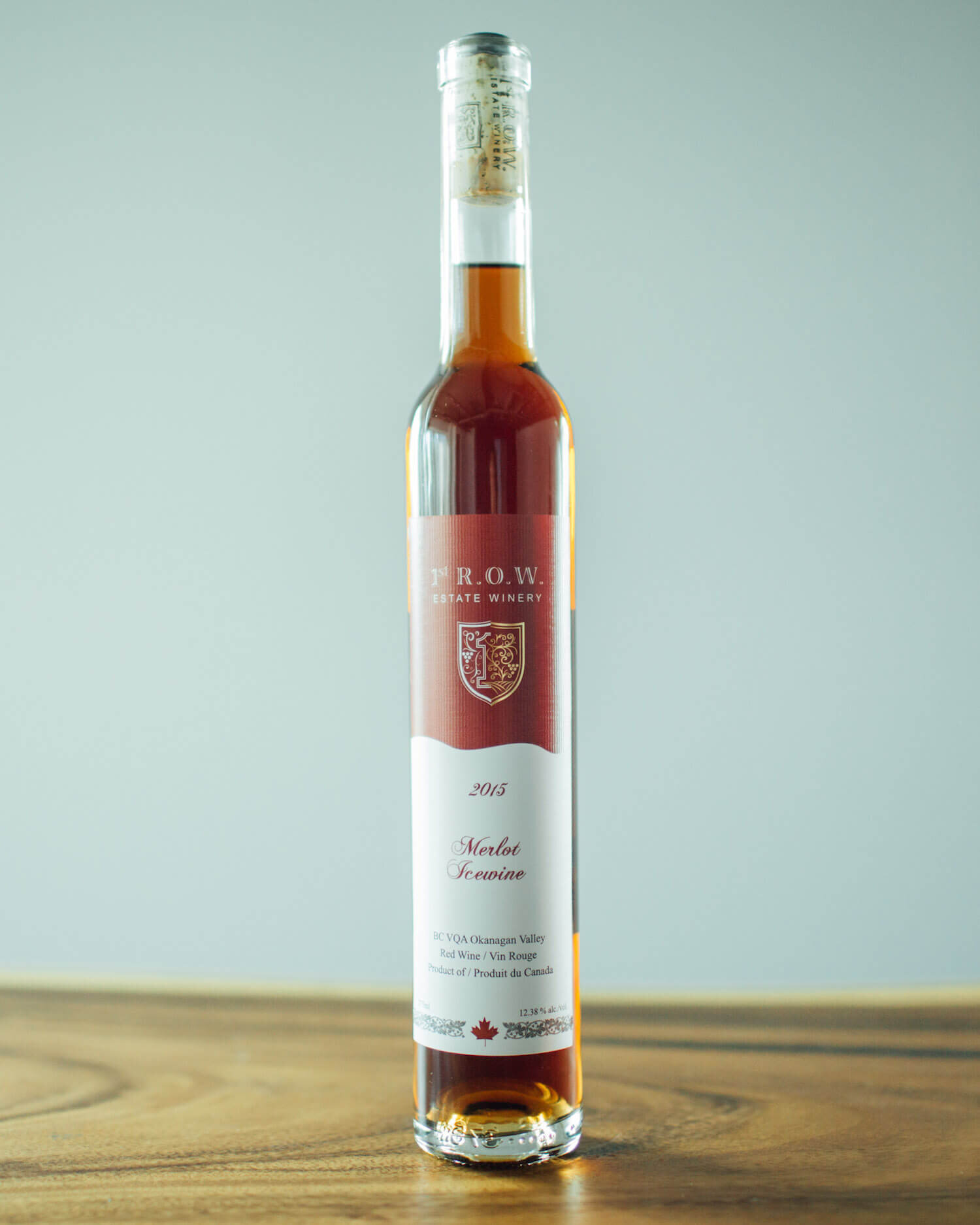This image features an unusual, elegant bottle of Merlot Ice Wine, distinctively long and narrow, resting on what appears to be an oak wooden table. The backdrop is a calming light green wall, creating a serene atmosphere that complements the dark, brownish hue of the wine within the bottle. The bottle is corked and adorned with a detailed label.

The label reads "First R.O.W. Estate Winery" at the top, followed by a shield emblem at its center, which contains an outline of a wand and intricate scroll work resembling grape plants. Beneath this, a white, curved banner prominently displays "2015 Merlot Ice Wine." Additional details on the label include "BCBQA, Okanagan Valley, Red Wine/Vin Rouge, Product of/Produit du Canada" and the alcohol content of "12.38%." At the bottom of the label, an oak leaf, signifying Canada, is bordered by a black line.